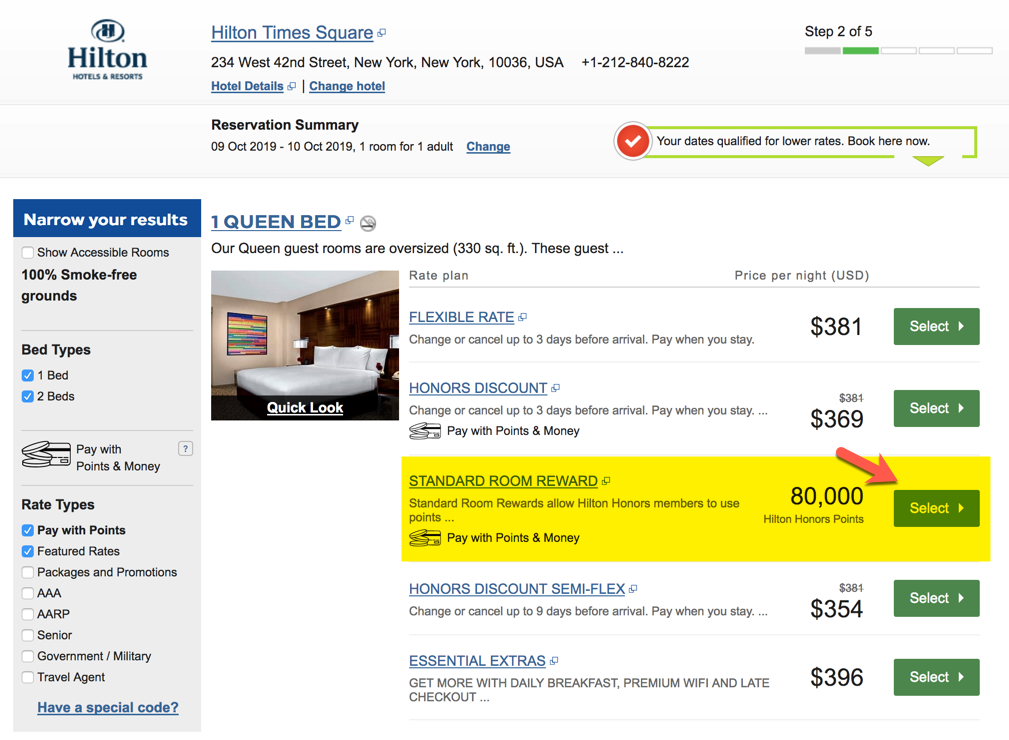A detailed reservation summary for Helton Hotels and Resorts at the Times Square location in New York City. The text includes the hotel address: 234 West 42nd Street, New York, NY 10036, USA. The reservation is set for one room for one adult, from October 9th to October 10th, 2019, with details mentioning various rates and options available. Narrow your results to show acceptable rooms which are 100% smoke-free, with options for one or two beds. Payment can be made with points or money, and discounts or packages like AAA, AARP, and senior government support are available. The guest rooms are oversized, approximately 330 square feet, and offer clean and comfortable accommodations. Cancellation policies vary: some options allow cancellation three days before arrival with payment due at the stay, while others offer semi-flexible cancellation policies up to nine days before arrival. The rates fluctuate from $354 to $396, with options for daily breakfast, premium WiFi, and late checkout for an additional fee. Honor members can redeem points, with standard room rewards costing 70,000 points.